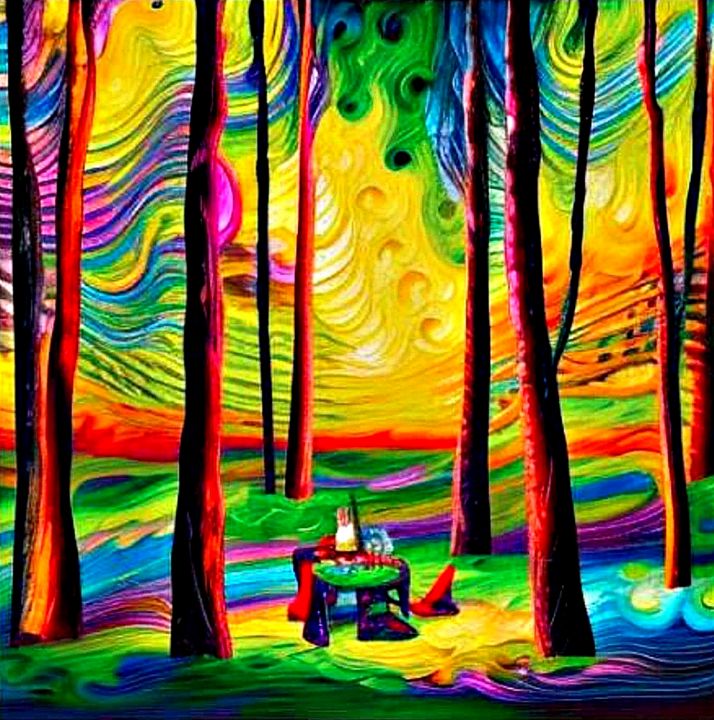This is an extraordinarily vivid painting brimming with intense colors and psychedelic patterns. The scene depicts a forest, but rather than showing foliage, it focuses on the tree trunks, which are bathed in an array of neon hues—reds, oranges, purples, and blues. These trees stretch upwards into a multicolored sky filled with swirling patterns of yellow, green, blue, and occasional red, creating a dynamic backdrop that almost appears oceanic. At the center of the image is a small table with a green tabletop and a possibly purple base, situated on what seems to be the forest floor, which is a whirl of green, purple, and yellow. It appears someone is seated at this table, and there’s a red wizard hat positioned to the right side. Light emanates from the table, casting contrasting shadows on the trunks of the trees and adding depth to the scene. The painting's eye-catching and surreal aesthetic, with its mixture of sharp contrasts and fluid swirls, gives it a distinctly trippy, fantastical feel.